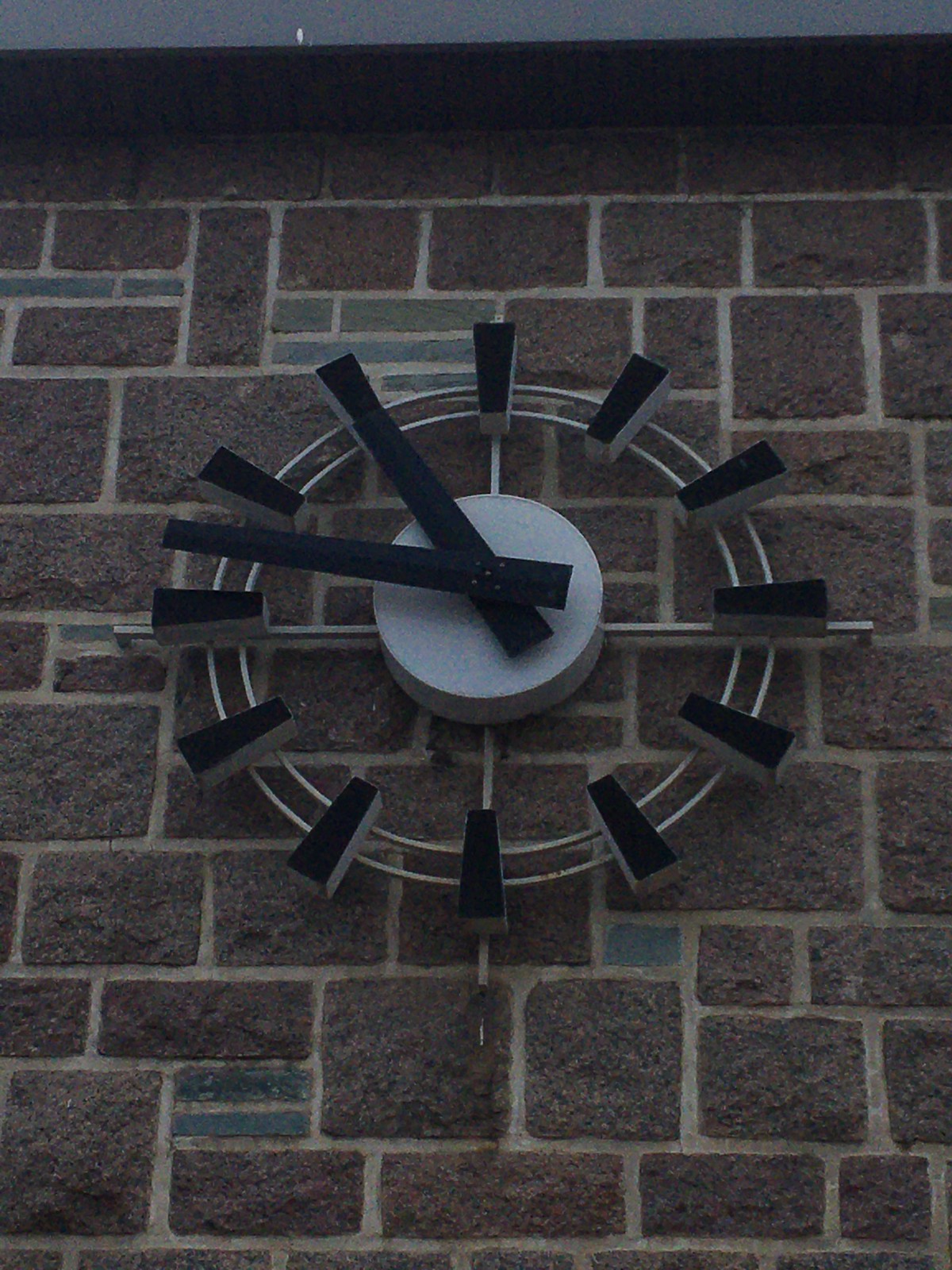This image features a unique, circular clock mounted on a meticulously crafted stone wall. The clock's design is characterized by two delicate metal rings that frame its minimalist yet striking face. Instead of traditional hour markers, the clock employs 12 small, black, three-dimensional blocks with silver sides, giving it a modern and edgy appearance. These blocks, distributed evenly around the clock, serve as indicators for each hour. At the center, a small, three-dimensional silver object anchors the clock's mechanism, adding an industrial touch. The clock is equipped with two short, square-shaped hands for hours and minutes, enhancing its contemporary design. Notably, the clock's back is entirely open, allowing a clear view of the wall it is affixed to. The wall itself is composed of grey stone blocks interspersed with occasional blue stones, creating a random yet aesthetically pleasing pattern that adds to the overall visual appeal of the installation.